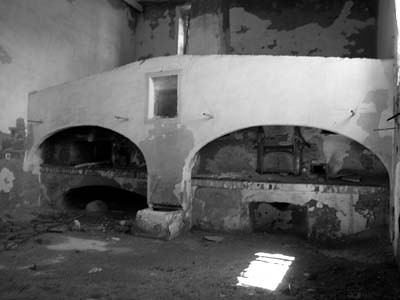This black-and-white photo captures the dilapidated interior of a building, possibly an abandoned industrial space or warehouse. The scene is dominated by two prominent archways with cylindrical structures emerging from above each. These archways frame what might have once been ovens or storage spaces. Centrally positioned between the arches is a rectangular window, partially round, through which sunlight streams, casting a bright rectangle of light on the gray concrete floor. The window is flanked by walls on either side and a larger wall behind, all exhibiting extensive chipping and peeling of what used to be white paint. Debris and grime litter the floor and the base of the archways, enhancing the sense of abandonment. Above the archways, additional pipes or poles protrude, possibly remnants of an industrial setup. The overall atmosphere is one of neglect and decay, accentuated by the stark black-and-white contrast that emphasizes the textures and deterioration of the space.